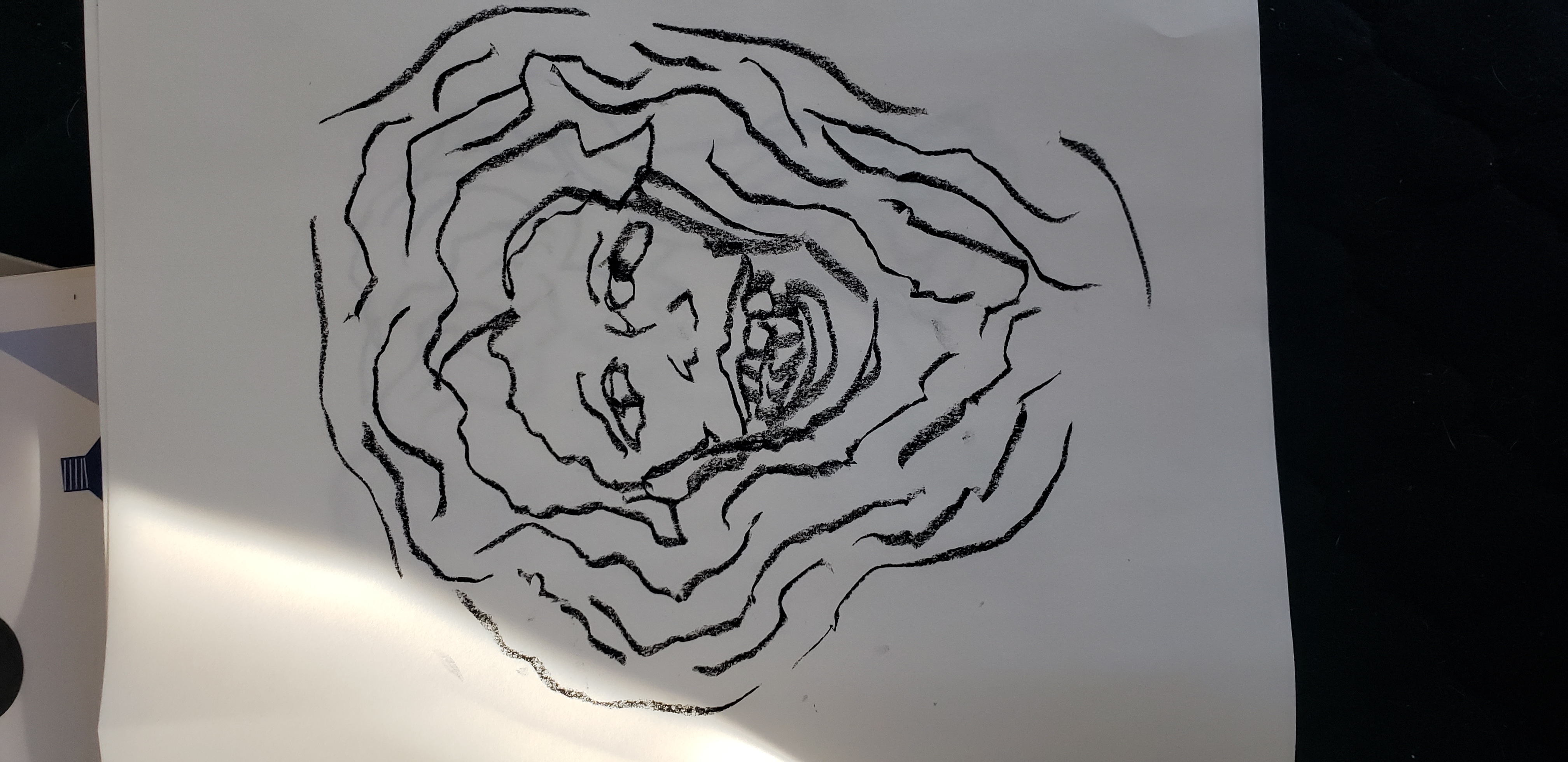A detailed and descriptive caption for the given image would be:

"A hand-drawn illustration seems to capture the chaotic essence of 'tweaker madness.' The central figure, depicted with exaggerated, jagged teeth and wide, manic eyes, bears a resemblance to characters from the classic cartoon 'Ren and Stimpy.' The teeth, reminiscent of cartoon characters biting rocks, are uneven and gap-filled, enhancing the character's frantic, unhinged appearance. Surrounding the figure is a flurry of black squiggly lines, symbolizing a background of madness and disarray. The drawing is rendered on white paper with dense black ink shading, particularly prominent on the right side of the image, lending a stark contrast. The surreal and wild imagery vividly brings to mind the zany, manic energy typical of 'Ren and Stimpy' animation."